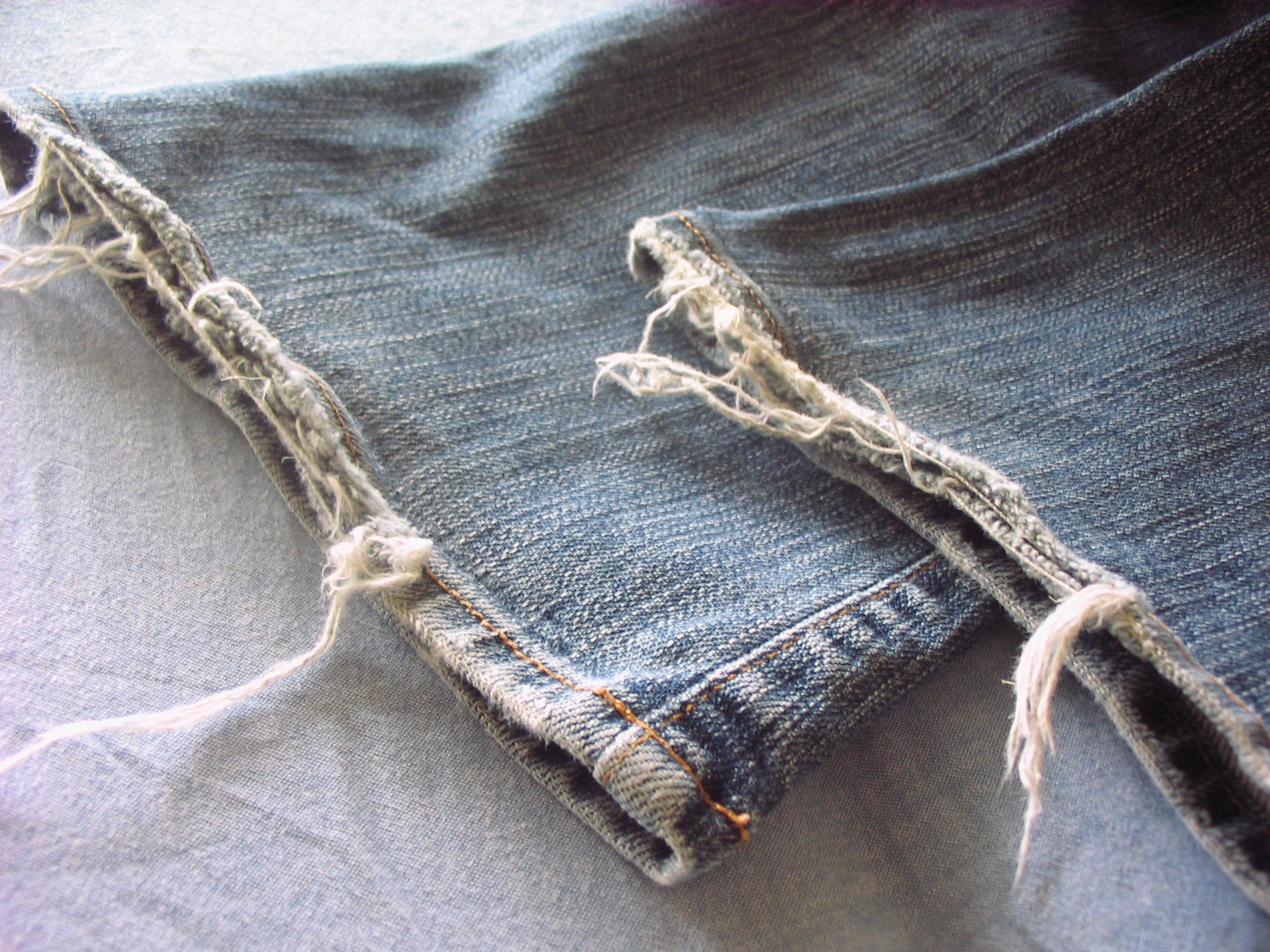This highly zoomed-in photograph captures the frayed bottom cuffs of a pair of dark blue, distressed jeans, neatly laid out on what appears to be a light gray or whitish piece of fabric. The background, which is some type of cloth covering a platform or bed, adds softness to the image. Visible are approximately the bottom six inches of the two pant legs. The left leg is more prominently featured, while the right leg is partially obscured. Both legs showcase light golden stitching at the seams and are heavily frayed at the ends, with white threads dangling irregularly, conveying a rugged, distressed-by-design look. The texture contrasts between the roughed-up edges and what appears to be otherwise relatively new denim adds depth and character to the image.